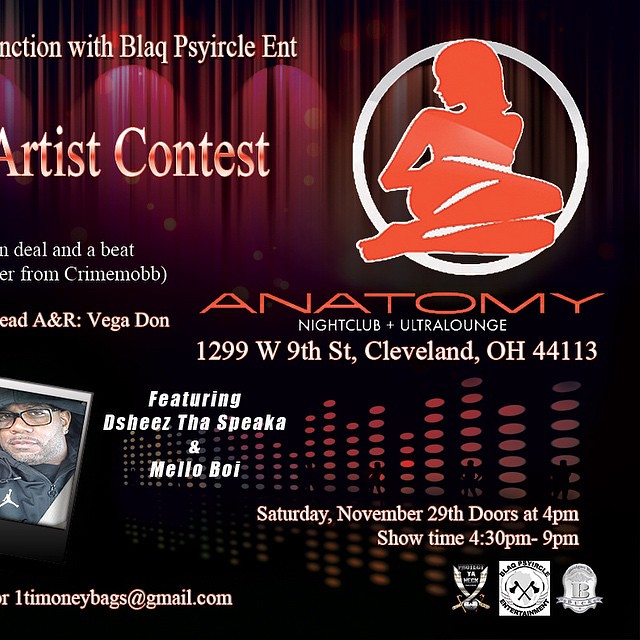The image is a poster or leaflet advertising an event at the Anatomy Nightclub Ultra Lounge located at 1299 West 9th Street, Cleveland, Ohio, ZIP code 44113. The prominent headline at the top, albeit partly obstructed, mentions Black Circle Entertainment and Artist Contest. The focal point is a white circle containing the silhouette of a seated woman with skin-toned shading, her knees drawn to one side. In bold red text, the word "Anatomy" stands out, followed by "Nightclub Ultra Lounge" beneath it. The event details are listed, announcing a show on Saturday, November 29th, with doors opening at 4 p.m. and performances scheduled from 4:30 p.m. to 9 p.m. Featured artists include Oshish, The Speakah, and Mellow Boy. 

To the left, there's partial text mentioning "Deal and a beat from Crime Mob" and the name Faye Goddard. At the bottom left-hand corner, there is a half-cut image of a black man wearing black-rimmed sunglasses, a trimmed beard and mustache, and a black coat with a basketball logo. A logo featuring the white circle and female silhouette is situated to the right side of the poster.